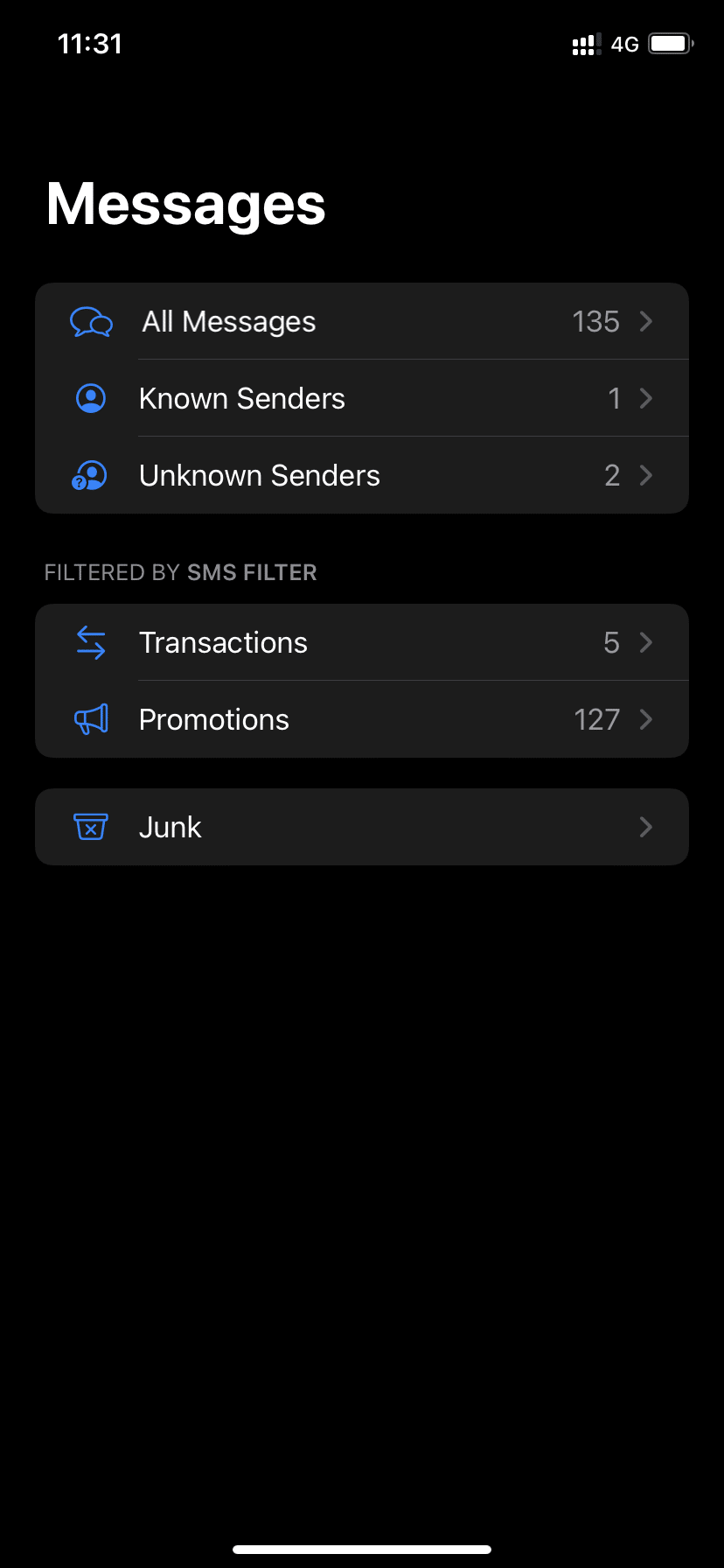This is a detailed screenshot from a messaging app on a cell phone, taken at 11:31, with a battery level of 99%. The background is black, and the text is white with blue icons. At the top, the app is labeled "Messages." Below, several drop-down menus can be seen:

1. **"All Messages"** – Accompanied by a blue word bubble icon on the left and the number "135" on the right.
2. **"Known Senders"** – Marked by a blue person icon with the number "1" on the right.
3. **"Unknown Senders"** – Labelled with a blue icon and the number "2" on the right.

In the second section, the label reads "Filter by SMS Filter" and contains additional drop-down menus:

1. **"Transactions"** – Featuring a blue icon of arrows going left and right, with the number "5" on the right.
2. **"Promotions"** – Displayed with a blue microphone icon and the number "127" on the right.
3. **"Junk"** – Represented by a blue trash can icon, with no accompanying number.

The interface is neatly organized, with a clear black-and-white aesthetic punctuated by blue icons for easy navigation.